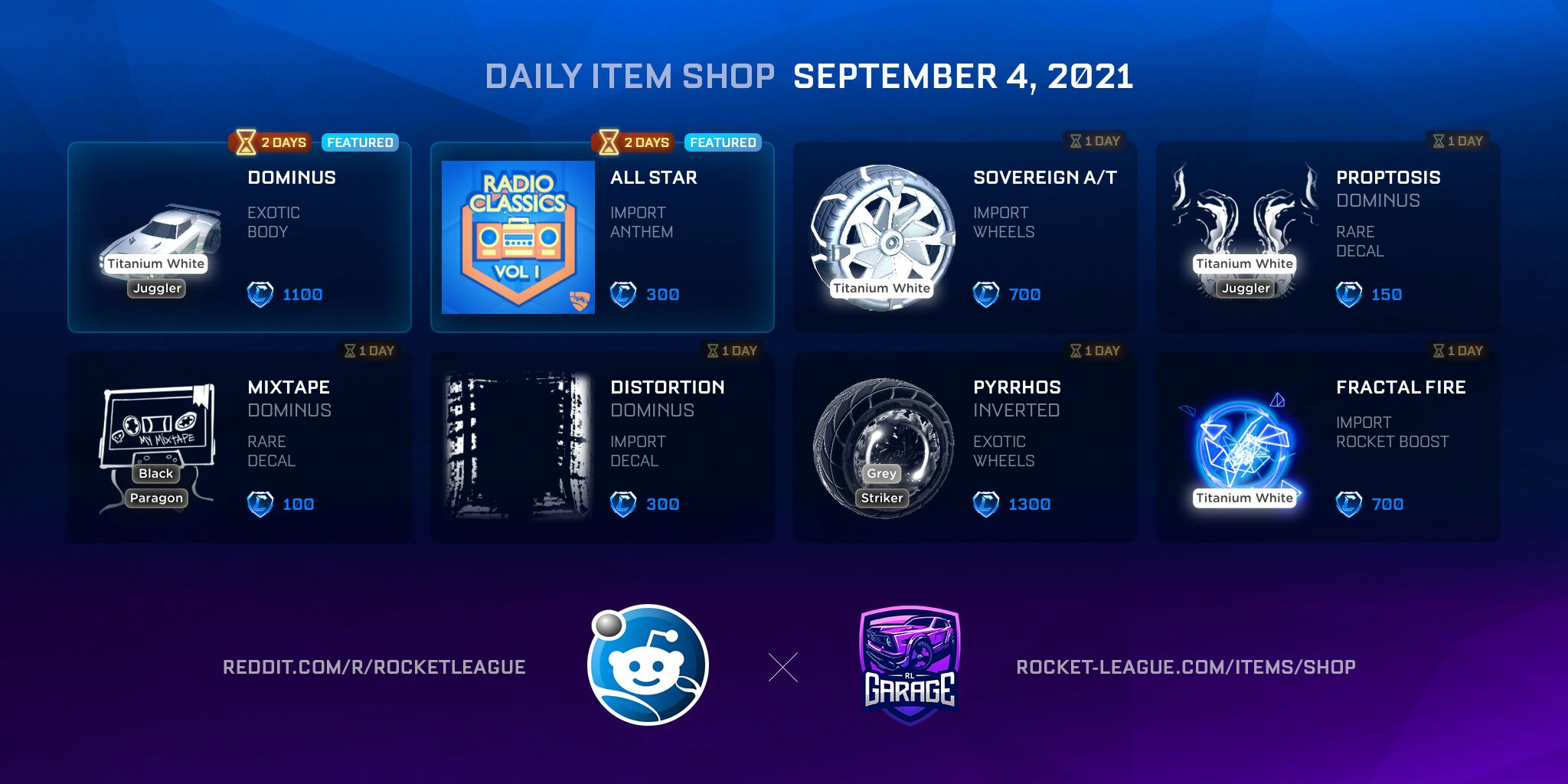The image is a screenshot from a video game, showcasing a vibrant background that features a gradient effect transitioning from blue at the top to various shades of purple at the bottom. The top portion of the background is predominantly blue, while the bottom section features a darker purple on the left side and a lighter purple on the right side. In the center, the blue and purple gradually blend into one another, creating an ombre effect.

At the very top of the image, there is light gray text that reads "Daily Item Shop," and to the right of this, white text displays the date "September 4, 2021." Below this header, there are eight distinct boxes arranged in two rows of four.

In the top-left box, white text reads "Ominous" accompanied by an image of a white car. To the right, the next box contains the text "All-star" and a small screenshot of what appears to be a game titled "Radio Classics," featuring a stereo. The third box from the left displays "Sovereign AT" with an image of a tire, and the rightmost box shows "Proptosis" along with a black and white image or symbol.

In the bottom-left box, directly beneath "Ominous," is the text "Mixtape" alongside a white computer. The box to its right contains the text "Distortion" and an image of a door with a completely black interior. Moving further right, the next box displays "Virus" next to an image of a black tire, and the far-right box features "Fractal Fire" accompanied by a blue triangular effect.

At the very bottom of the image, there is a purple icon to the left that looks like a collaboration logo. Initially, it appears to be the Discord logo, but on closer inspection, it is revealed to be the Reddit logo instead.